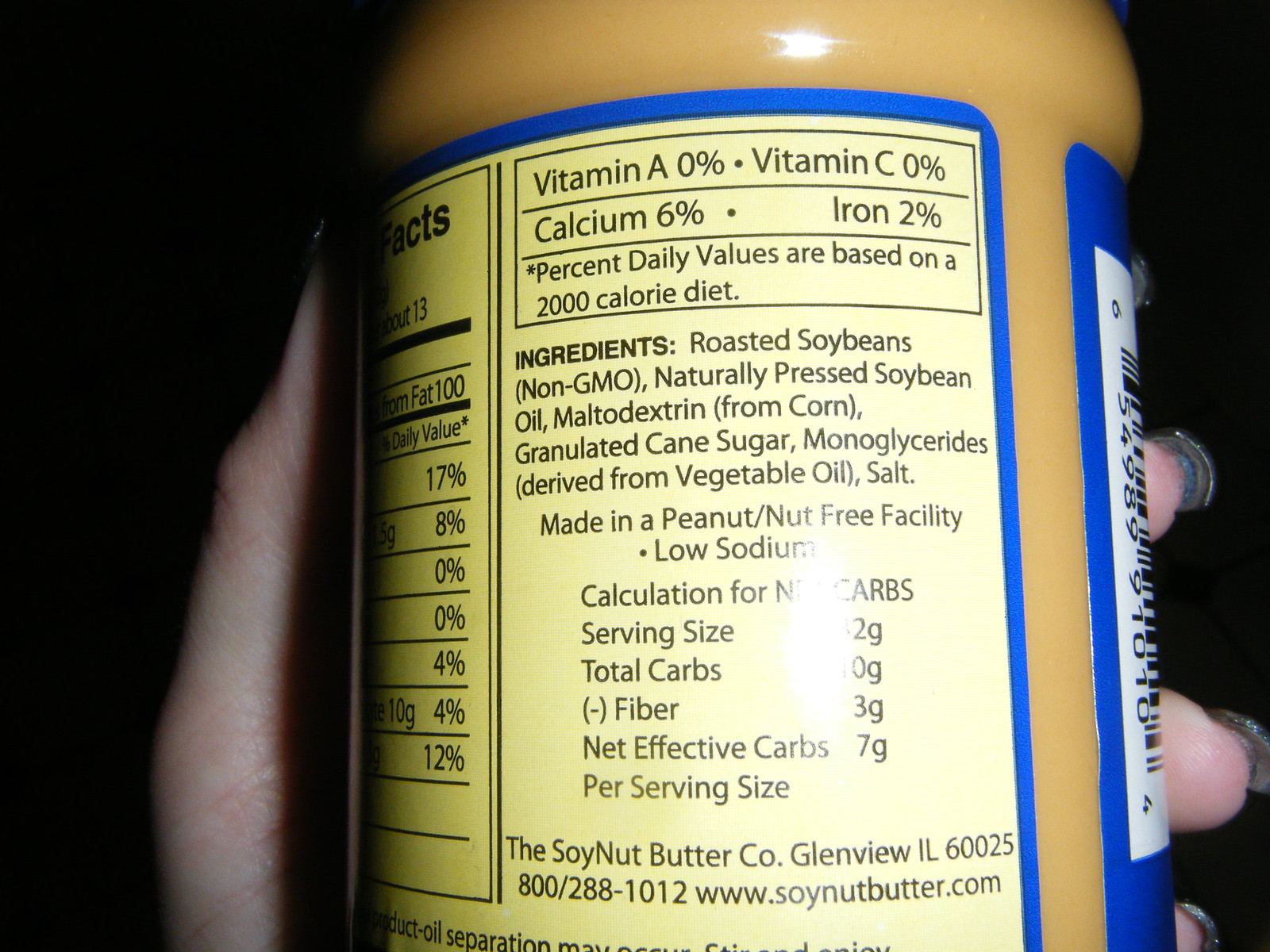This image is a close-up of a jar of soy nut butter from the Soy Nut Butter Company, based in Glenview, Illinois. The jar has a light brown substance inside and is flanked by black areas. On the left side, a thumb is visible gripping the jar, while on the right side, fingers with silver-tipped fingernails are wrapped around it. The label on the back of the jar is partially visible, with a blue border and nutritional facts such as vitamin A and C percentages, and a list of ingredients including roasted soybeans, naturally pressed soybean oil, maltodextrin, granulated cane sugar, monoglycerides derived from vegetable oil, and salt. The product is made in a peanut-free facility. Additional details on the label include serving size, carbohydrate content, company information, and a partial QR code on the far right side.